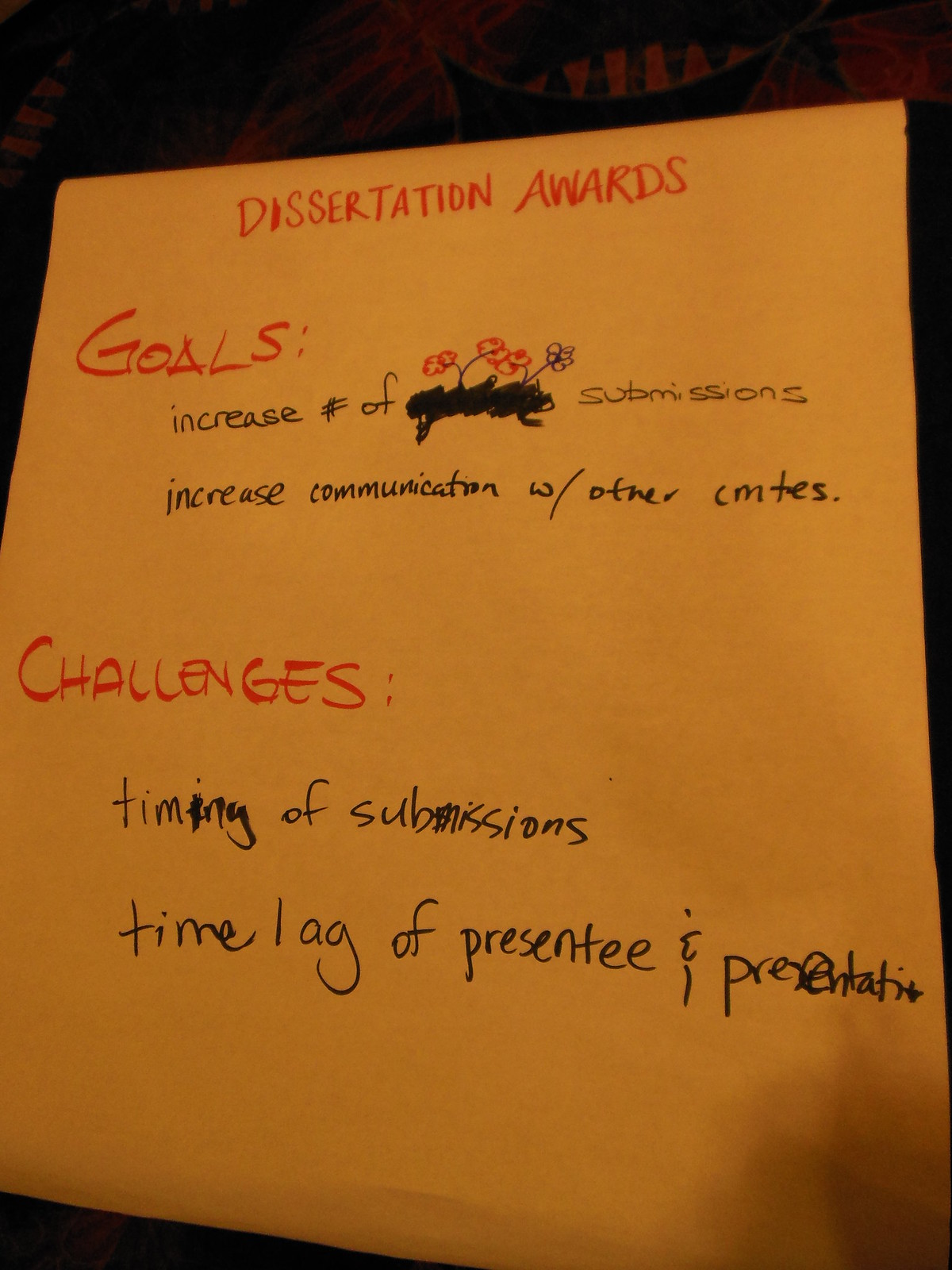The image shows a close-up of a slightly wrinkled, yellow notepad page with handwritten notes. At the top of the page, "Dissertation Awards" is written in red felt pen. Below that, in red and on the left side of the paper, "Goals:" is prominently marked. Following this in black ink, the notes state, "Increase number of submissions" and "Increase communication with other CMTES." Further down, again in red ink, "Challenges:" is highlighted in large letters, followed by bullet points in black writing: "Timing of submissions" and "Time lag of presentee and presentation." The background of the image is black and there is a brown smudge in the bottom right corner of the paper. The handwriting appears hurried and imprecise, with some doodles and scribbles interspersed among the text.